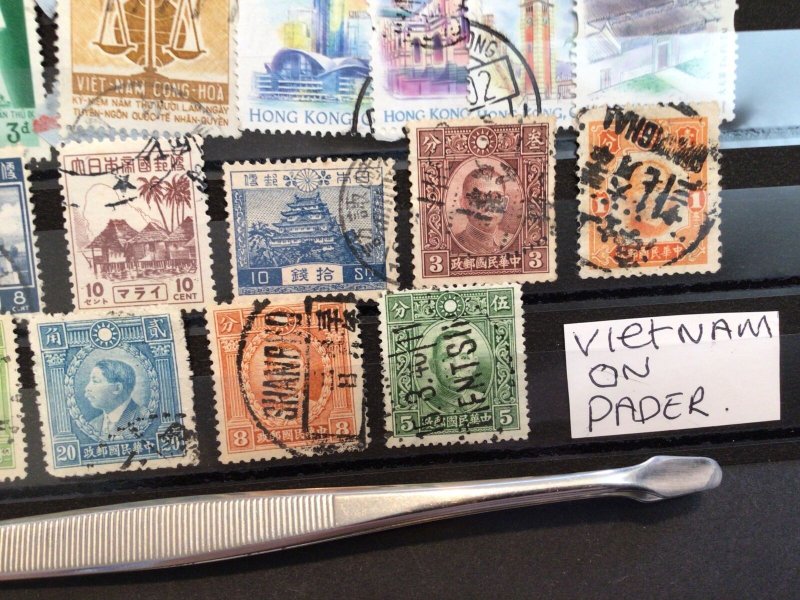This detailed photograph captures a portion of a meticulously arranged stamp collection. The stamps, which vary in color from blue, orange, green, red, to burgundy, are neatly organized in three rows on a black-tiered rack with transparent strips holding them securely in place. The top row features four stamps, the middle row five, and the bottom row three. Each stamp is denominated with values ranging from 3 to 20 cents, suggesting they may be historical or collectible stamps, possibly even forms of old currency. A closer inspection reveals stamps from different regions, most prominently Vietnam, Hong Kong, and Singapore, each showcasing vivid imagery, including famous personalities and traditional structures such as castles and village huts.

In the bottom right corner, a small piece of paper labeled "Vietnam" indicates the primary focus of the collection. Adjacent to this, a silver metal instrument resembling a pair of tweezers, designed for handling the delicate stamps, underscores the careful curation of the collection. Some stamps bear postmarks, adding to their authenticity and historical value. This photograph provides a captivating glimpse into a personal, well-organized assembly of international stamps, with a predominant emphasis on Vietnamese philately.